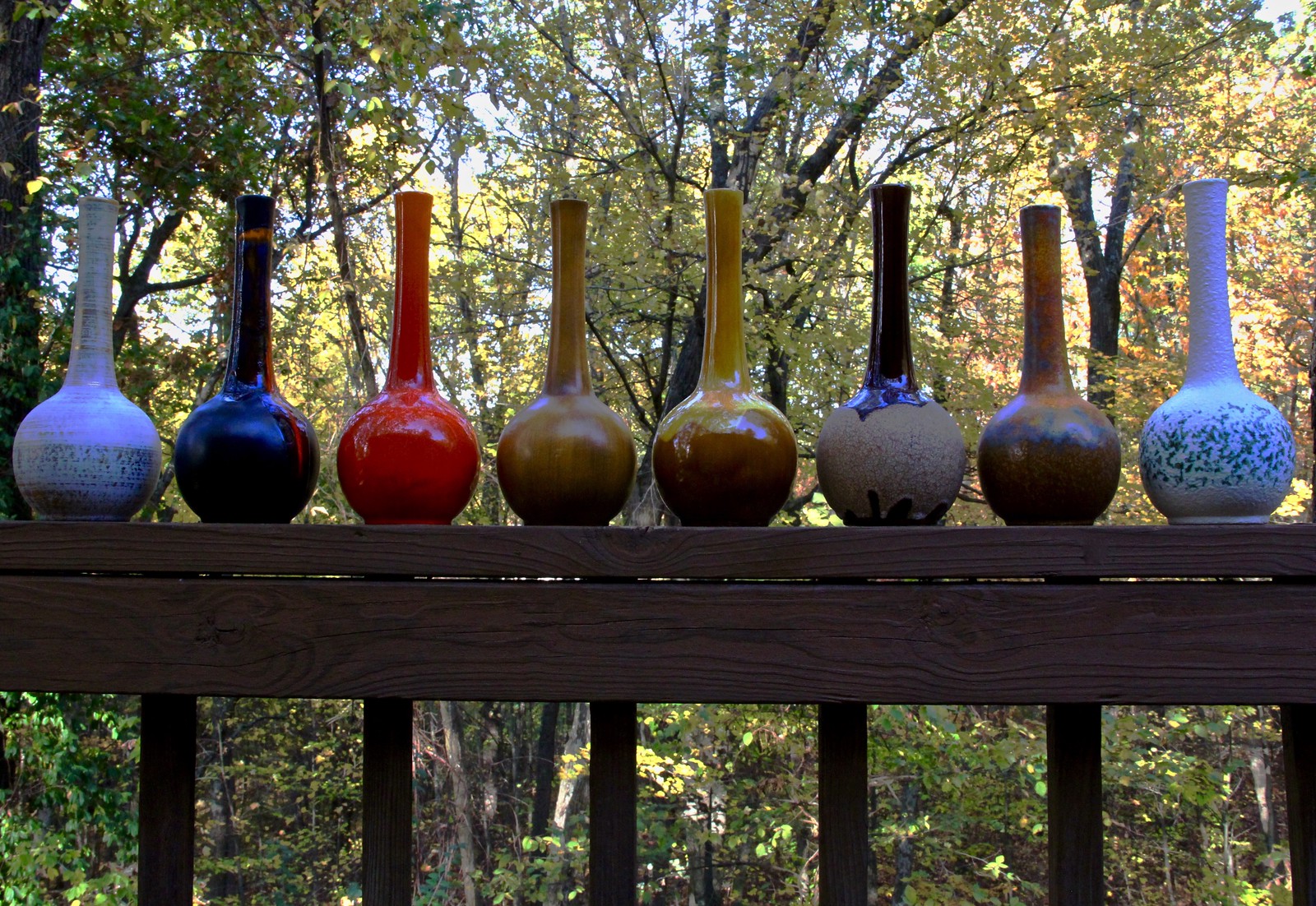This color photograph captures a serene outdoor scene, focusing on a series of eight beautifully crafted pottery vases meticulously lined up along the handrail of a wooden deck. The deck, likely situated on the second story, features a dark wood stain on its flat top rail and vertical 2x2 pickets. The top rail has an L-shaped design, and together with the pickets, it frames a stunning natural backdrop of dense woodland, where the tops of trees display a mix of vibrant autumn leaves and verdant greens against a visible sky.

The vases are uniform in shape but diverse in their colors and finishes. Each vase boasts a spherical or globe-shaped bottom that gracefully tapers into a tall, slender neck, approximately eight inches in height. From left to right, their colorful array begins with a vase having a gray base transitioning into a white-dipped neck. Next is a black vase accented with red glaze striping, followed by a striking cherry red vase. The fourth vase showcases a greenish-brown glaze, while the fifth exhibits a yellowish-brown hue. The sixth vase stands out with its raw stoneware body, marked by a black-glazed foot and neck. The seventh vase may be salt-fired, given its characteristic brown sheen. Finally, the last vase features a matte white glaze adorned with subtle greenish speckles around its belly.

This orderly arrangement of vibrant vases against the dark wooden rail and the lush woodland beyond creates a visually stunning tableau, blending man-made artistry with the natural beauty of the outdoors.